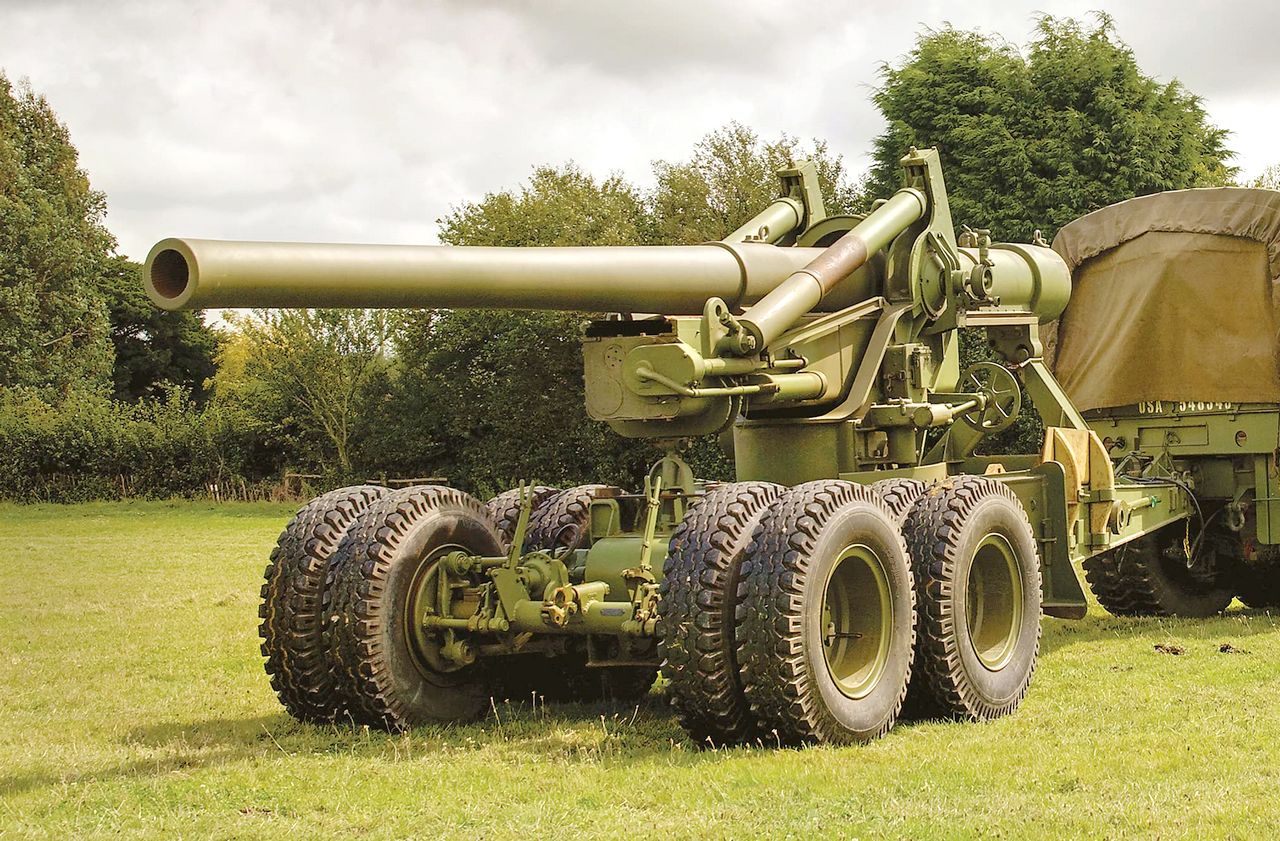This is a highly detailed, professional photograph featuring a very large missile launcher situated on a trailer with eight heavy wheels. The trailer and missile launcher, all painted in olive-green army colors, are being towed by a Jeep marked with "USA" and some identifying numbers. The main focus of the image, aside from the launcher, is its long, narrow, high-powered barrel and the complex array of mechanisms for its operation. The Jeep is partially covered by a brown tarp. The setting is a rural field with grass underfoot and a backdrop of trees and bushes against a gray-blue sky suggesting impending rain, although the image is illuminated by sunlight. This outdoor scene is crisply captured, emphasizing the large, robust equipment amidst the natural surroundings.